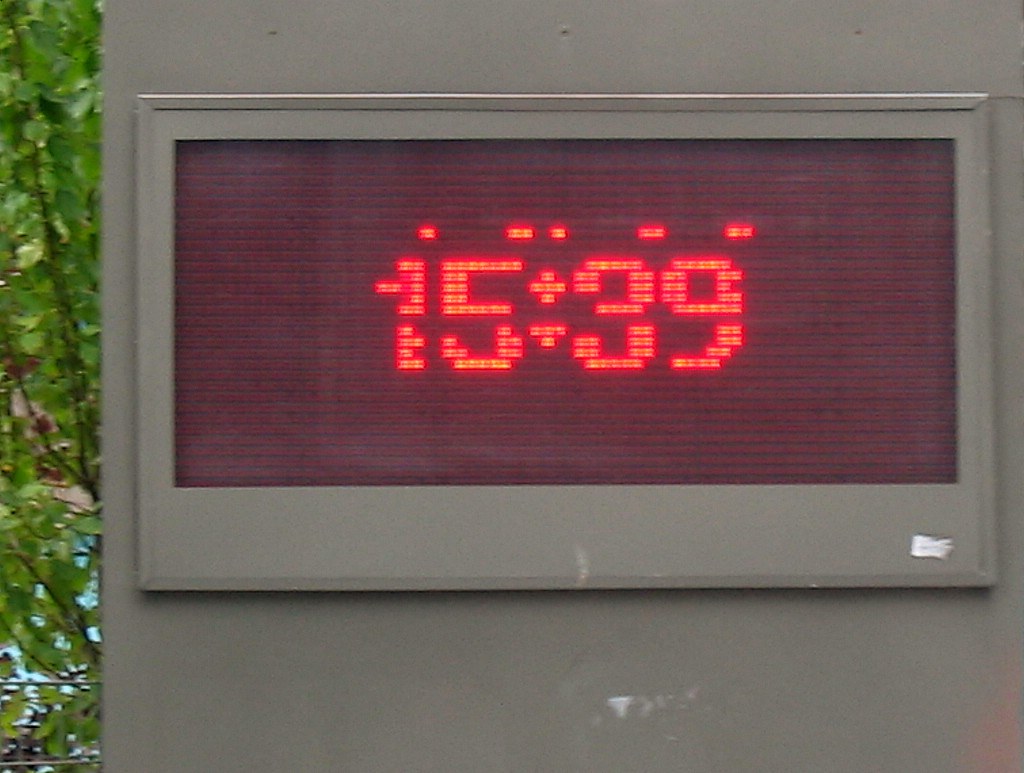This photograph captures a red digital clock affixed to the side of an outdoor sign for a building, the business name of which remains unidentified due to the framing of the image. The clock, which reads "15:39" (or 3:39 PM), is positioned beneath the cropped section of the sign's outer edges, which are gray. In the background, lush green bushes provide a natural contrast to the man-made elements. The lower right corner of the sign bears a word in white, although the image's slight blurriness leaves it illegible. Notably, the clock appears weathered, likely from prolonged exposure to sunlight, resulting in some stray illuminated bulbs above the numbers "1539."